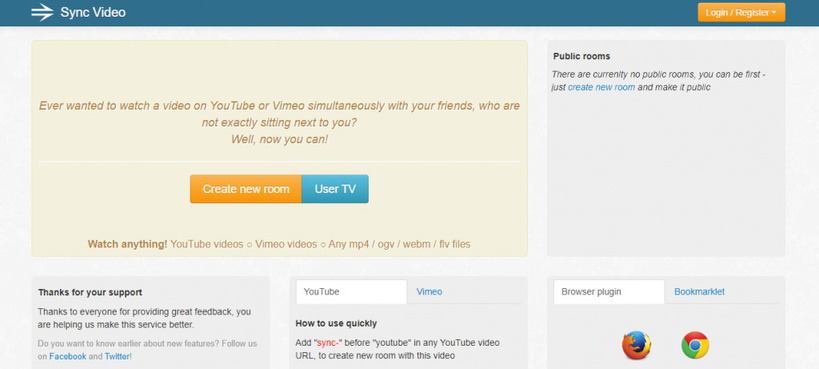Screen capture of a website interface viewed on a computer monitor. At the top of the page, there is a dark green navigation bar with two right-facing arrows and the text "Sync Video" on the left-hand side. In the upper right corner, there is a prominent rectangular orange button labeled "Login/Register" in white text.

Below the navigation bar, the background shifts to a slightly yellowish section, containing a promotional message that reads: "Ever wanted to watch a video on YouTube or Vimeo simultaneously with your friends who are not exactly sitting next to you? Well, now you can." Directly beneath this text are two rectangular buttons: one orange and one blue, both featuring white text.

Continuing downward, a darker orange bold header states: "Watch anything YouTube videos, Vimeo videos, any MP4, OGV, WebM, and FLV files." 

At the bottom of the page, there is a gray section. On the left side, in bold black text, it says: "Thanks for your support." On the right side, there is a search box with the white text "YouTube" inside it, accompanied by the word "Vimeo" in blue text to its right. Below the search box, a bold heading in black reads: "How to use quickly."

In the bottom right corner of the screen, within another gray area, is a white bar labeled "Browser Plugin" with the word "Bookmarked" in blue text to its right, followed by two icons: the Firefox icon on the left and the Chrome browser icon on the right.